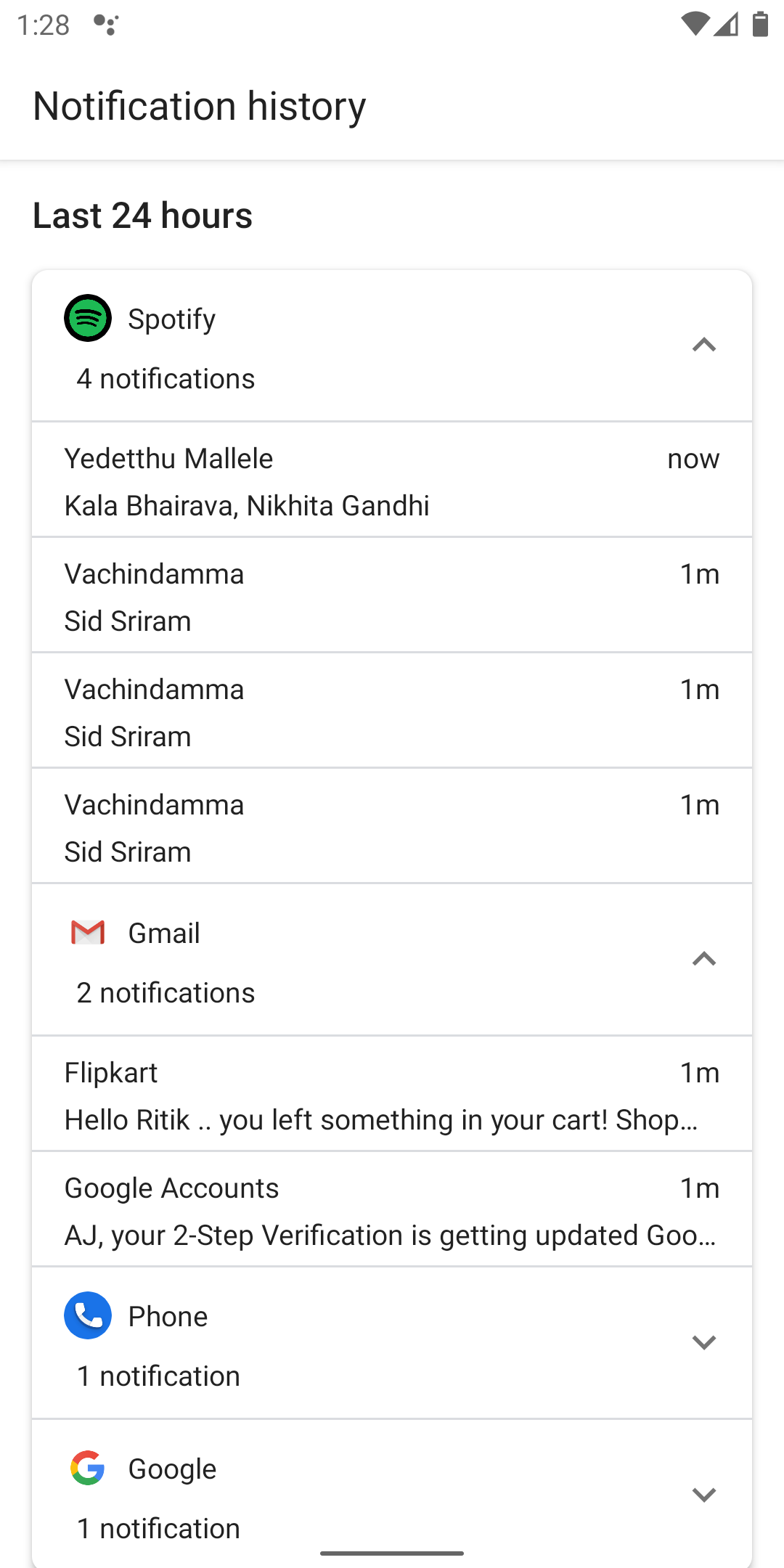A screenshot of a smartphone screen displaying the time as 1:28, along with battery life and signal reception icons. The primary title of the screen is "Notification History," with a subheading of "Last 24 hours." The main section features a boxed window containing several rows of notifications. 

The first row shows a Spotify notification with the distinct Spotify logo. Below it, there are several rows listing the names Yadethu Malele, Kala Bhairava, and Nikita Gandhi, indicating recent notifications labeled as "now."

Further down, three consecutive rows list the name Vachindama Sridharam, all marked as notifications from "one minute ago." Following this, a Gmail row indicates two notifications. One is from Flipkart, stating, "Hello, Riddick, you left something in your cart," also from "one minute ago." Another Gmail notification mentions, "AJ, your two-step verification is getting updated," under the header of Google accounts.

The section concludes with a single notification row from the Phone app and another from Google, each summarizing one recent notification.